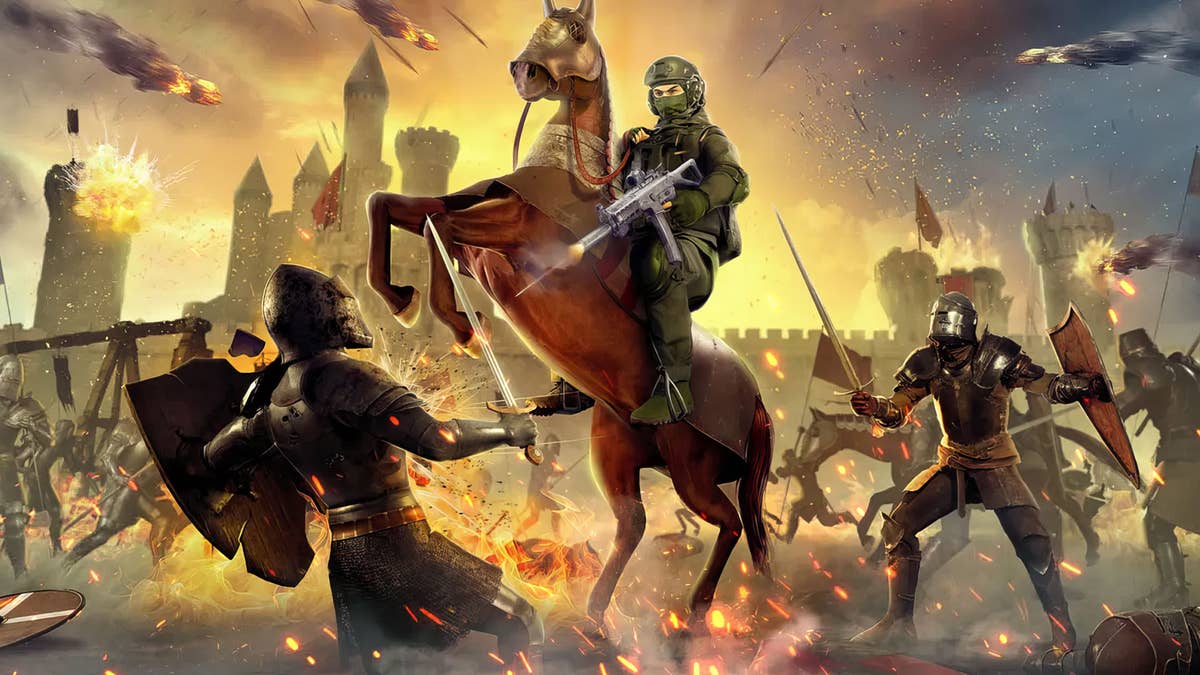This image depicts a highly detailed and dramatic battle scene with 3D, realistic qualities reminiscent of artwork or a video game. The landscape is chaotic with numerous elements of fire, flames, and smoke, making the sky appear as though it's filled with fireworks. Central to the composition is a horse rearing up on its hind legs, armored and ridden by a soldier in modern army gear, who is actively shooting a machine gun. This modern soldier is targeting a knight clad in full medieval armor with a sword, located to the left of the picture.

Surrounding them, numerous other knights in armor, equipped with shields, swords, and traditional weapons, are engaged in fierce combat. The backdrop features a gray, bombed-out castle that still has portions preserved, adding to the historic versus modern contrast. The sky above the castle is mostly cloudy and smoky, with a small patch of blue peeking through in the upper right. Fireballs and arrows are shown mid-flight, with explosions visible where cannonballs have struck the castle, suggesting intense action and turmoil throughout the scene. The image vividly blends elements of medieval and modern warfare, creating a thrilling and dynamic portrayal of a time-bending battle.